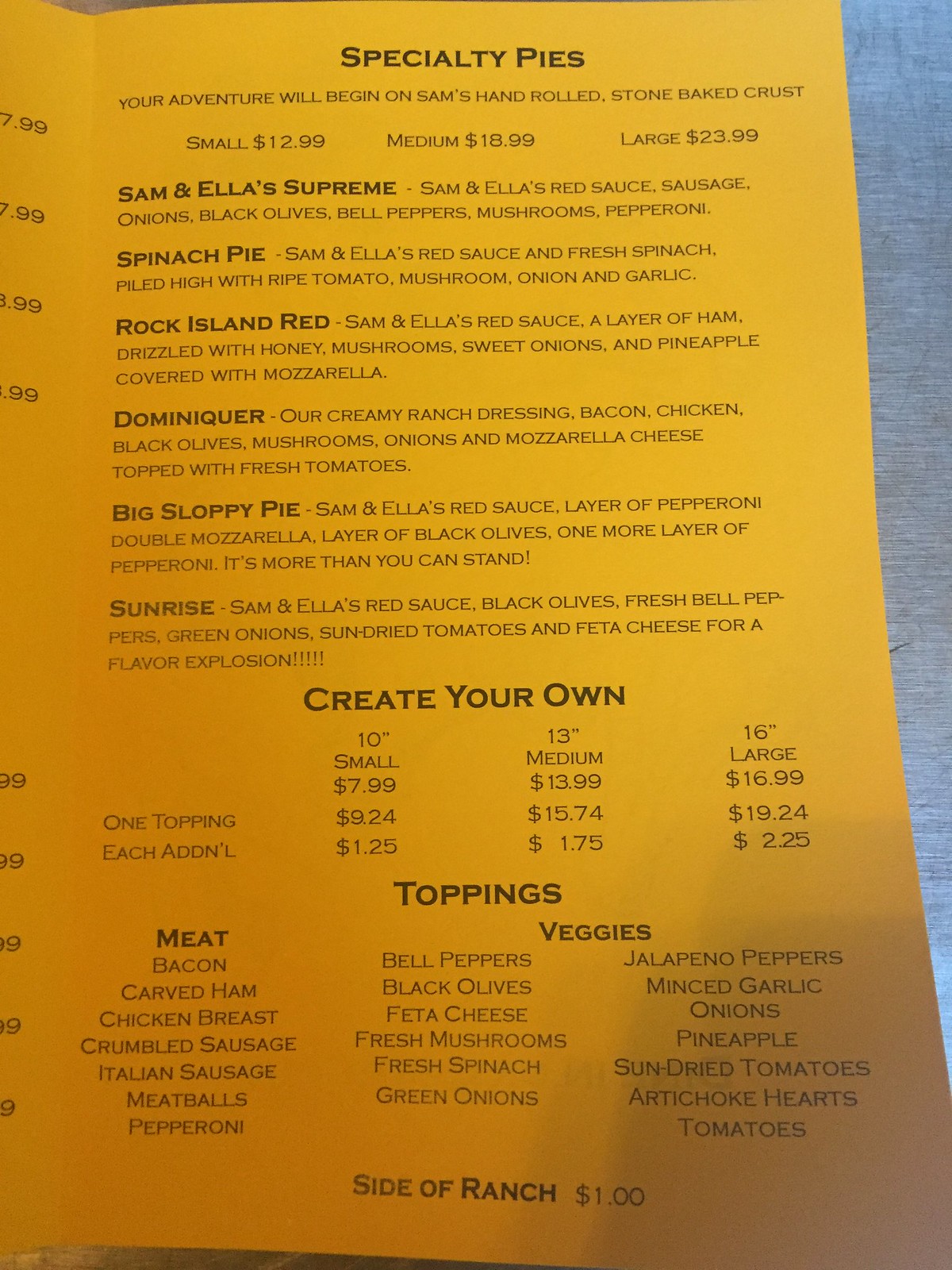**Caption**

The image captures the right side of an open menu set against a worn-down, scratched surface, with the main focus on the yellow-colored menu featuring black text. At the very top center of the menu, bold letters announce "Specialty Pies." Below, in all capital letters but not bold, it reads, "Your adventure will begin on Sam's hand-rolled stone baked crust." There are three size options listed: Small $12.99, Medium $18.99, and Large $23.99.

Following that, six specialty pie options are detailed, each with a bold, black title in capital letters. The first option, "Salmonella Supreme," includes a list of ingredients: "Salmonella's red sauce, sausage, onions, black olives, bell peppers, mushrooms, pepperoni." Next is "Spinach Pie," described with "Salmonella's red sauce, fresh spinach piled high with ripe tomato, mushroom, onion, and garlic."

"Rock Island Red" features "Salmonella's red sauce, layer of ham drizzled with honey, mushrooms, sweet onion, and pineapple covered with mozzarella." Another option, "Dominique," lists "creamy ranch dressing, bacon, chicken, black olives, mushrooms, onions, and mozzarella cheese topped with fresh tomatoes."

At the bottom, the menu presents an option to "Create Your Own" with three size choices: 10-inch, 13-inch, and 16-inch large, with one topping included and additional toppings available, divided into meat and veggie categories across three columns. Lastly, the bottom center notes a side of "Cider Ranch $1." The black text on the yellow paper is clearly printed, creating a striking visual contrast.